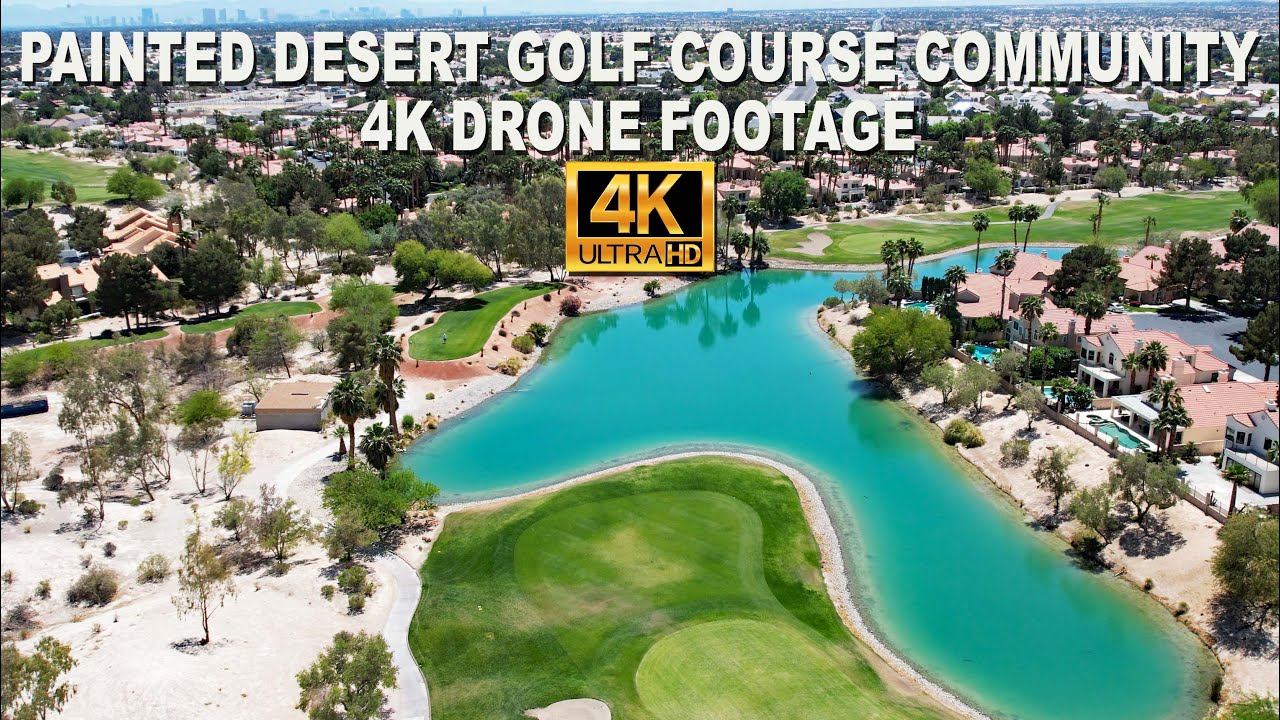This aerial photograph captures the picturesque Painted Desert Golf Course Community on a clear, sunny day. The centerpiece of the image is a uniquely T-shaped, blobby pond with aquamarine water, featuring a thicker bottom section and a top that is broader on the left and narrows to the right. Surrounding the pond, the lush, green grass of the golf course contrasts against a white sandpit on the left, dotted with scraggly bushes and trees. The left side of the photograph also showcases a desert landscape. In the top half of the image, houses and additional foliage are visible, while to the right, buildings with pools in their yards punctuate the scene. The overall palette combines the greens of trees and foliage with the pink and green hues of building rooftops. At the top of the photograph, white capital letters spell out "Painted Desert Golf Course Community," followed by the centered text "4K drone footage." Below this, outlined in a gold rectangle within a black square, is the label "4K Ultra HD."